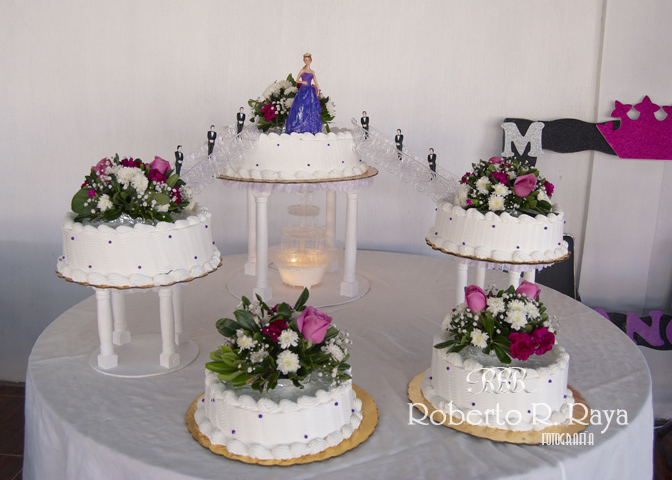This photograph features a grand, intricately designed cake display reminiscent of 1980s wedding or Sweet 16 celebrations. Centered on a round table draped with a white tablecloth, the display boasts a total of five round, single-layer cakes adorned with white icing and elegant floral decorations, including white flowers, pink buds, and red roses.

The focal point is the tallest cake positioned in the middle at the back, elevated on white columns and adorned with a figurine of a woman in a long, formal purple gown and a tiara. Flanked by two smaller cakes on medium-high stands, each connected to the central cake by clear plastic stairways featuring tuxedo-clad male figurines, this central piece creates a harmonious visual flow. Two additional cakes are directly placed in front of the display on the table, each mirroring the floral theme.

Details such as the possible decorative use of gold-plated plates under some cakes, a non-functional but visually striking fountain beneath the tallest cake, and a black decorative strip in the background further enhance the celebratory ambiance, suggesting a feminine-themed occasion.